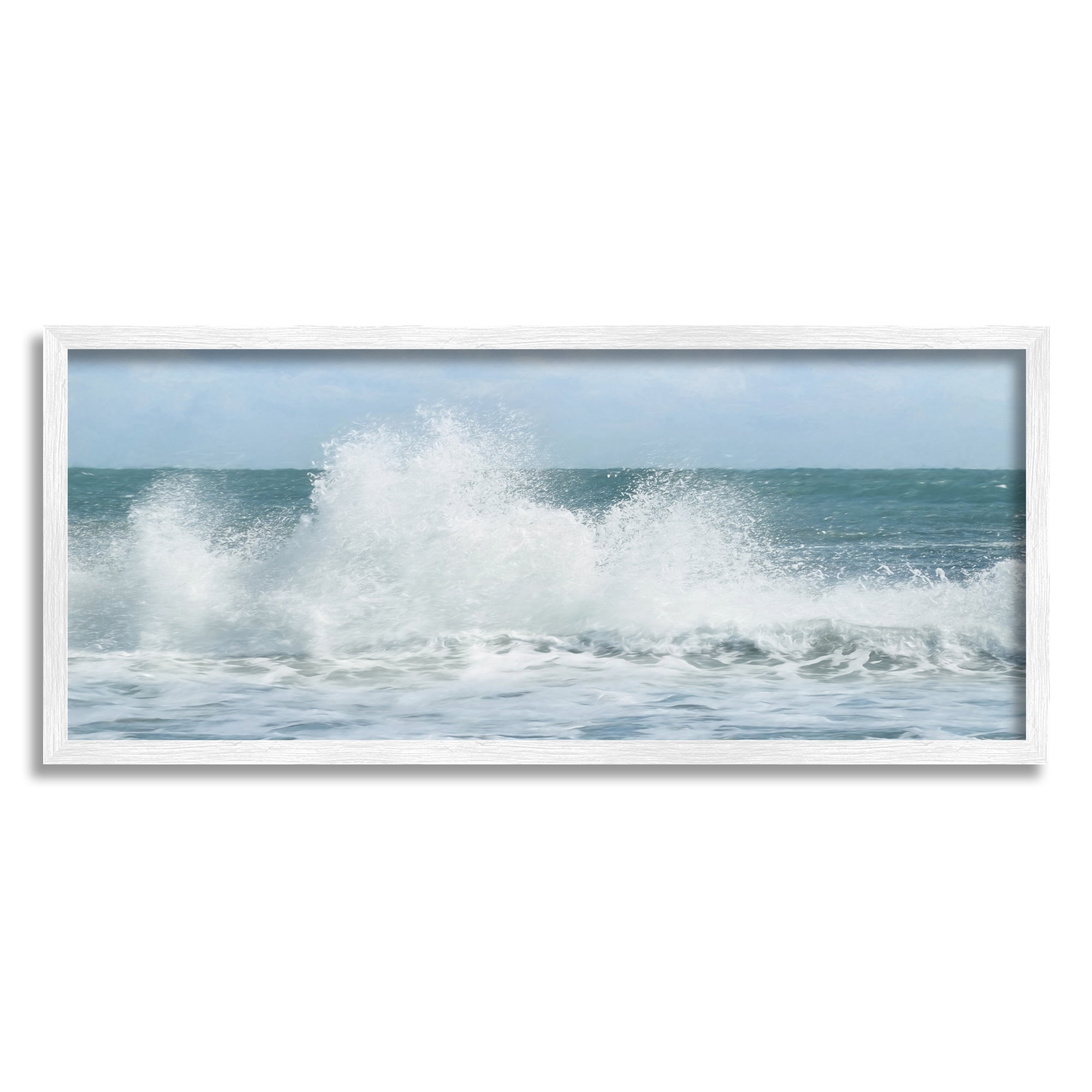In this hyper-realistic photograph, a dynamic seascape captures the raw power and beauty of ocean waves crashing against a rocky outcrop. Encased in a white wooden picture frame set against a minimalist white backdrop, the image vividly portrays waves transforming into a cascade of foam as they collide with the rugged surface. The center of the photo highlights the waves turning white, breaking into countless smaller droplets and creating significant oxygen bubbles, a clear indicator of the water's activity. The scene is divided into contrasting elements: the turbulent, foamy white waves in the foreground and the comparatively calm, green-blue ocean in the background. Above, a serene light blue sky further emphasizes the contrasting energies of the scene below, making the image both visually striking and intricately detailed.